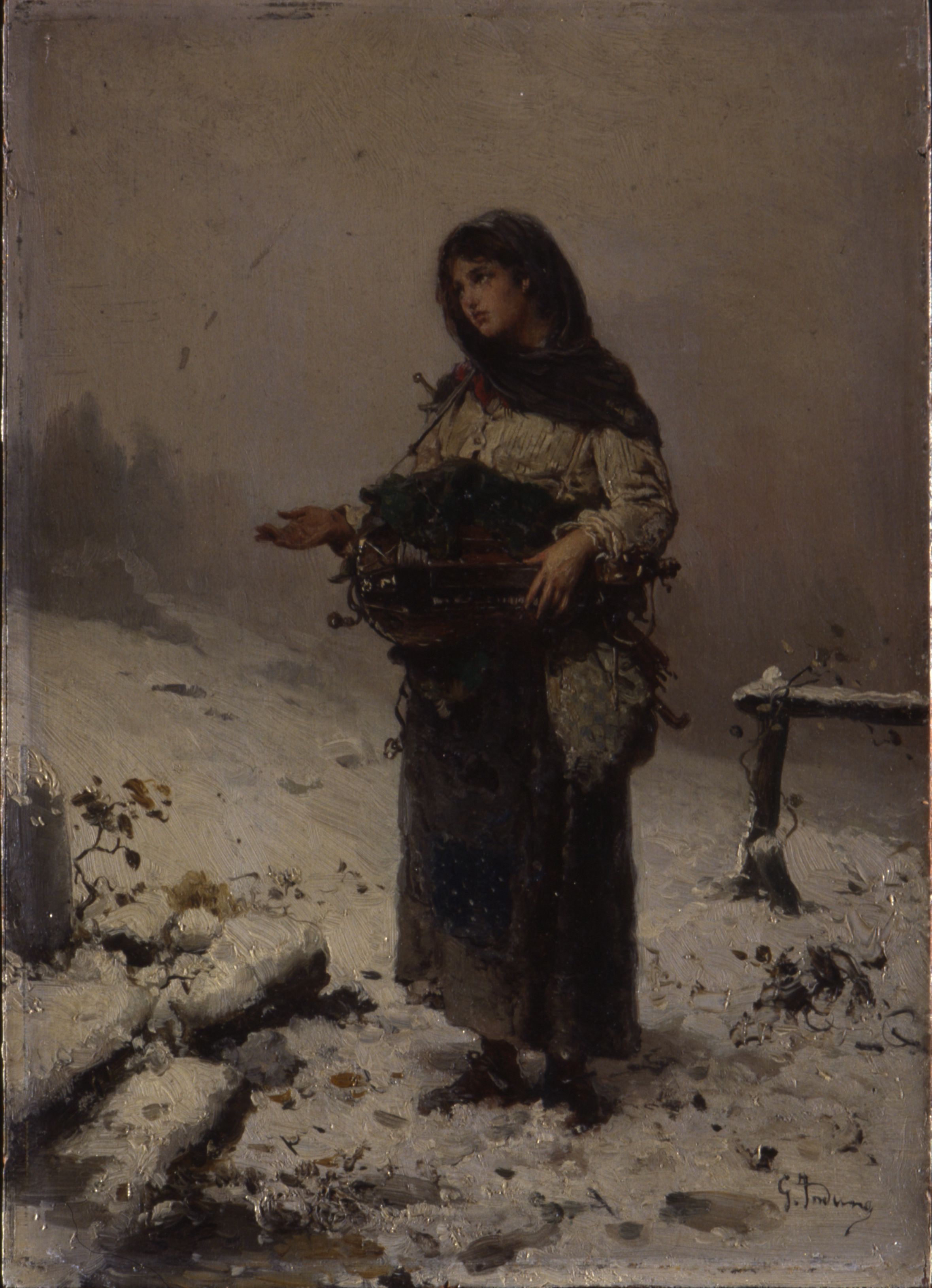In this portrait-oriented painting, a young woman, likely in her late teens or early 20s, stands alone on a snow-covered ground under a dark, foggy sky, hinting at twilight or night. Dressed warmly in heavy winter clothes, she wears a long heavy skirt that reaches her ankles, revealing dark shoes. Her white long-sleeved top is complemented by a scarf wrapped around her head, covering her ears and hair, with a flash of red at the neckline. 

She carries a cumbersome basket strapped over her shoulder, filled with items that could be bundles of firewood. Her left arm cradles the basket, while her right hand is extended in an upward cupping motion, as if she is waiting to receive something. The sparse, wiry plants breaking through the snow and the foggy silhouettes of trees in the background add to the stark, cold atmosphere.

The woman's expression is serious and somber, evoking a sense of loneliness heightened by the absence of other people. The overall color palette of the painting is very gray and dull, reinforcing the bleak, cold winter setting. The bottom right corner of the painting is signed by the artist.